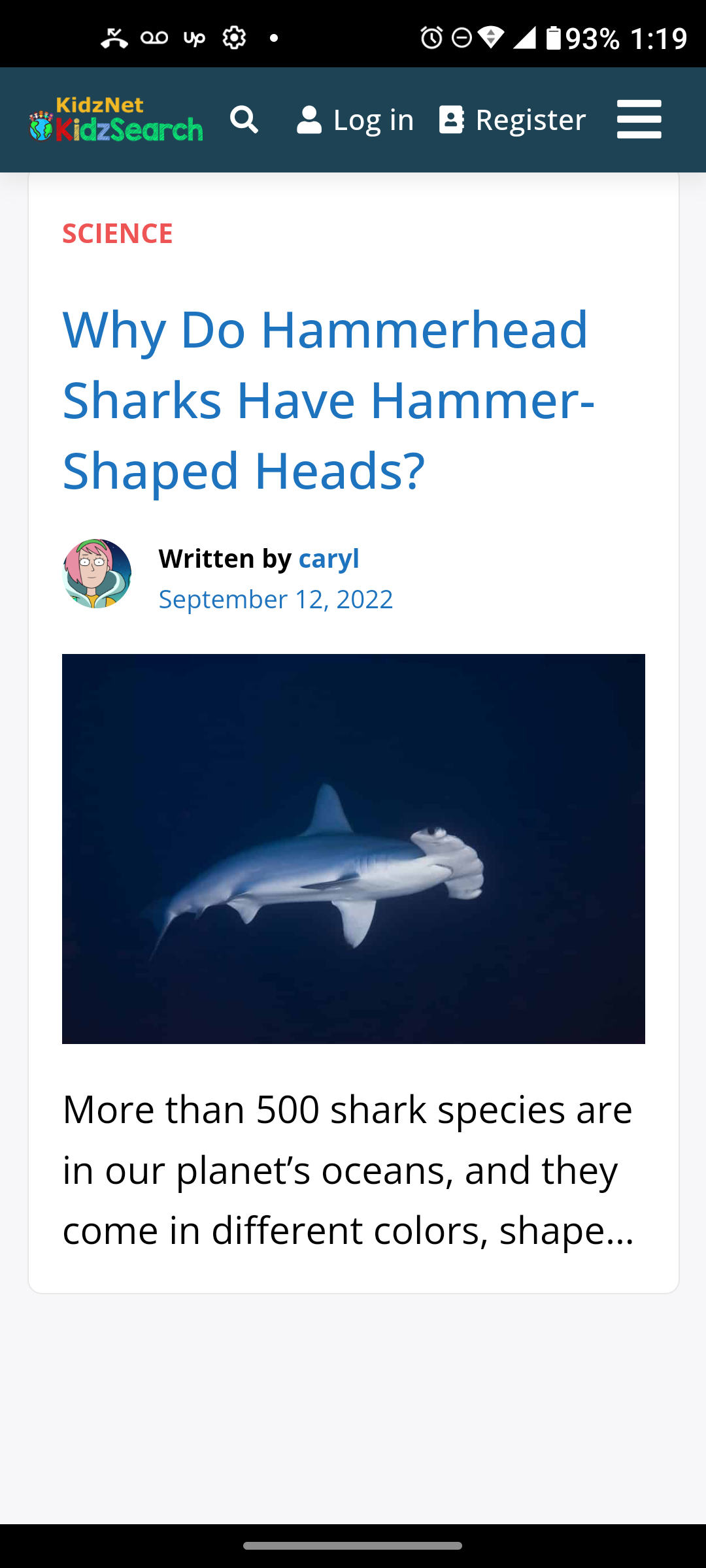A portrait-mode screenshot features a web page with a variety of elements. At the top of the image, there's a black stripe running across the upper left and upper right corners. In the upper left corner, there's an icon resembling a hung-up phone. The upper right displays the battery status, indicating 93% charged, next to the number 1:19.

Below this, the page transitions into a teal background on its left side. Here, the logo for "Kids Net Kids Search" is prominently displayed, consisting of a globe with children standing on it. Accompanying the logo, from left to right, are a search icon, a person icon labeled "Log In," and an address book icon labeled "Register," followed by three horizontal white lines that likely represent a menu.

The remainder of the page has a white background. Near the top left corner, the word "Science" is prominently highlighted in red. Below it, a teal heading poses the question, "Why do hammerhead sharks have hammer-shaped heads?" 

Adjacent to this heading is a cartoon avatar of a female with red, possibly pink, hair. The avatar represents the article's author, "Caryl," whose name appears in teal, likely as a live link. Below the author's name, the publication date "September 12th, 2022" is displayed.

Dominating the center of the screenshot is an image of a hammerhead shark, facing right with its fins and tail visible against a dark blue background. Below this image, text informs readers that "More than 500 shark species are in our planet's oceans, and they come in different colors and shapes."